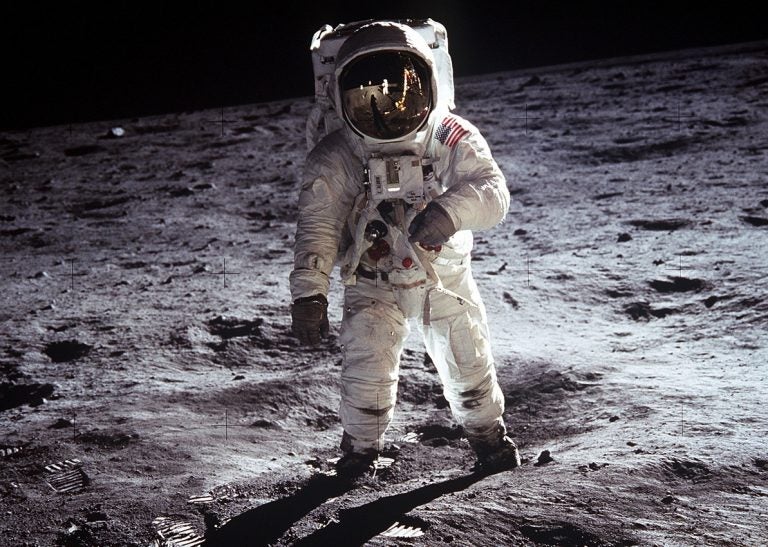This iconic photograph captures astronaut Buzz Aldrin on the chalky gray lunar surface during the historic Apollo 11 mission. Wearing a white survival suit adorned with a U.S. flag patch on his left shoulder, Aldrin is seen with gray gloves and boots, as well as a large oxygen pack and regulators strapped to his chest. His visor is down, reflecting the barren, rocky landscape of the moon, including small craters and numerous footprints. Within the visor's reflection, one can see Neil Armstrong, the first man on the moon, taking the photograph, along with the Apollo lander and a standing lamp illuminating the scene. The sky above the moon's horizon is pitch black, devoid of stars, emphasizing the stark, otherworldly environment. Aldrin's suit shows signs of lunar dust, particularly around his knees, adding to the authenticity and historic significance of this early astronaut photo.